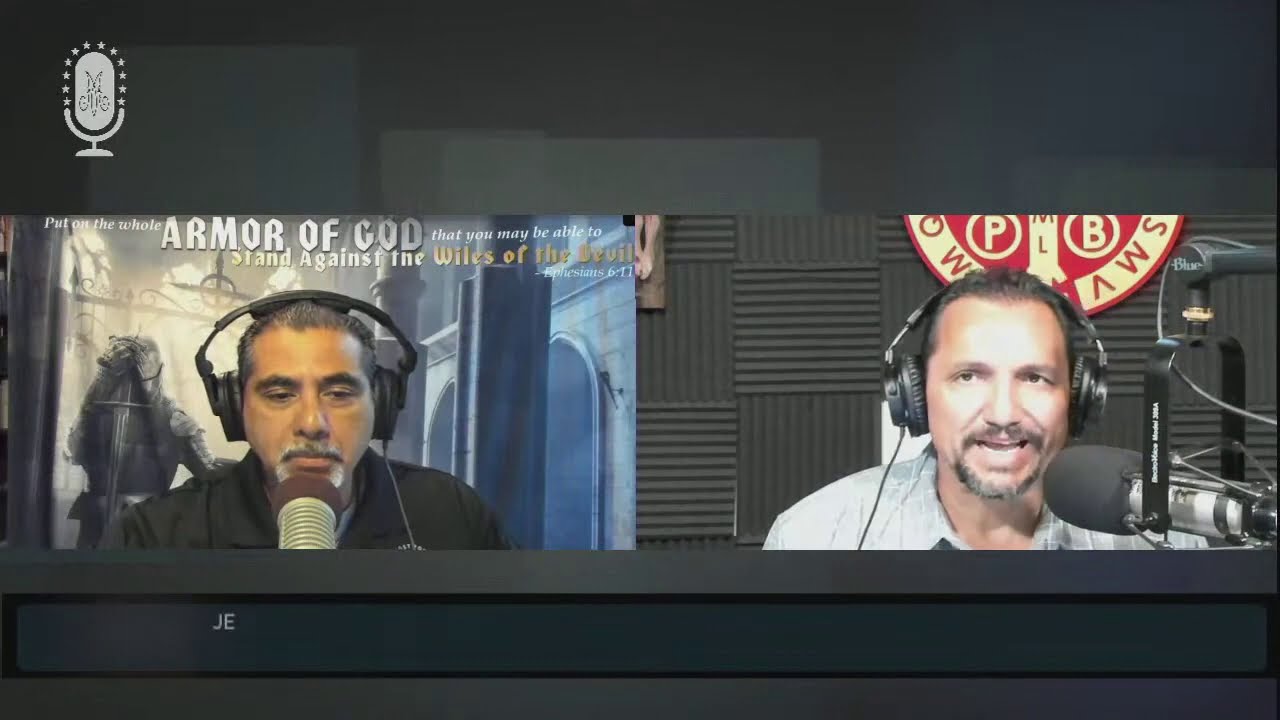This detailed image appears to be a color screenshot from a TV or computer, displaying a webcast or podcast in a landscape layout with a black and charcoal grey background. In the upper left corner, there is a grey microphone emblem. The screen is divided into two sections, each featuring a man wearing black headphones and speaking into a black microphone.

The left side showcases a man with salt-and-pepper hair, a goatee, and a black polo shirt. Above him, there's a prominent white text header stating, "Put on the whole armor of God that you may be able to stand against the wiles of the devil." The text 'armor of God' is capitalized and silver, while 'put on the whole' and 'that you may be able to' are in an italicized serif font. 'Stand against the wiles of the devil' is in gold. Behind him, a medieval-themed background features a knight or holy warrior figure with a sword set against a cathedral-like environment with a banner.

The right side features another man with brown hair and a mustache-goatee combination, wearing a grey collared shirt. This man is captured mid-sentence, and behind him, grey acoustic tiles are visible, with part of a red and gold sign displaying the letters 'P B'. A black band at the bottom of the image has the letters 'J E' toward the left side.